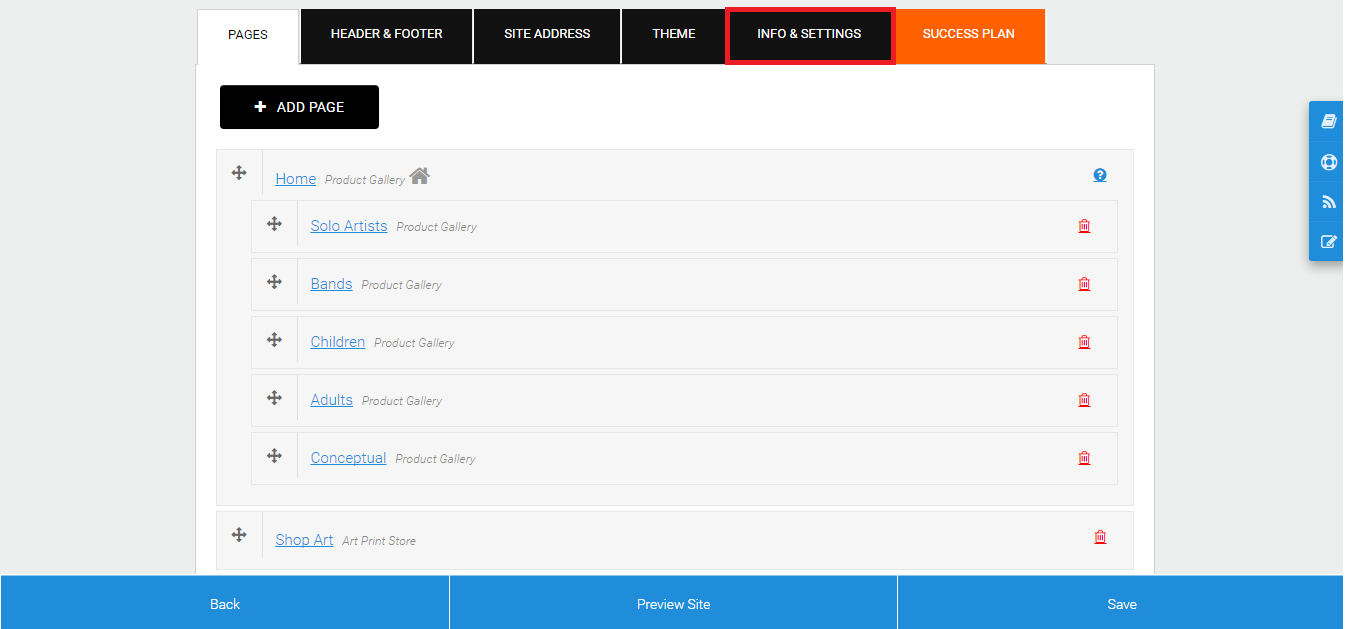The image depicts a highly detailed and annotated user interface screen. The layout is as follows:

- On both the left and right sides, there are grey areas.
- On the right-hand side, about a quarter of the way down, a section with a blue background features various icons: a book, a circle with a square inside it, Wi-Fi signal strength, and a piece of paper with a pencil on it.
- At the bottom of the screen, there are large buttons in blue text on a white background. These buttons, which occupy about a third of the screen each, are labeled "Back," "Preview Site," and "Save."
- At the top of the screen, there is a section labeled "Pages" in white text on a black background. Below this, there are three tabs in black text on a white background: "Header and Footer," "Site Address," and "Theme." These tabs are surrounded by a red border for some reason.
- Additionally, there is an orange text on a white background labeled "Success Plan."
- Beneath this section, there is a white button with black text labeled "+ Add Page."
- A grey section features a small, multi-directional arrow icon, with seven instances displayed in a row.
- Below this, there are several blue and grey underlined links, categorized as follows:
  - "Home" (underlined)
  - "Protect Gallery" (grey)
  - "Solo Artist" (underlined in blue)
  - "Protect Gallery" (grey)
  - "Bands, Product Gallery" (blue)
  - "Children" (blue), followed by "Product Gallery" (grey)
  - "Adults" (blue), followed by "Product Gallery" (grey)
  - "Conceptual" (blue), followed by "Product Gallery" (grey)
  - "Shop Ads" (blue), followed by "Product Gallery" (grey)
  - "Art Print Store" (grey)

This concludes the layout description of the user interface screen in the image.